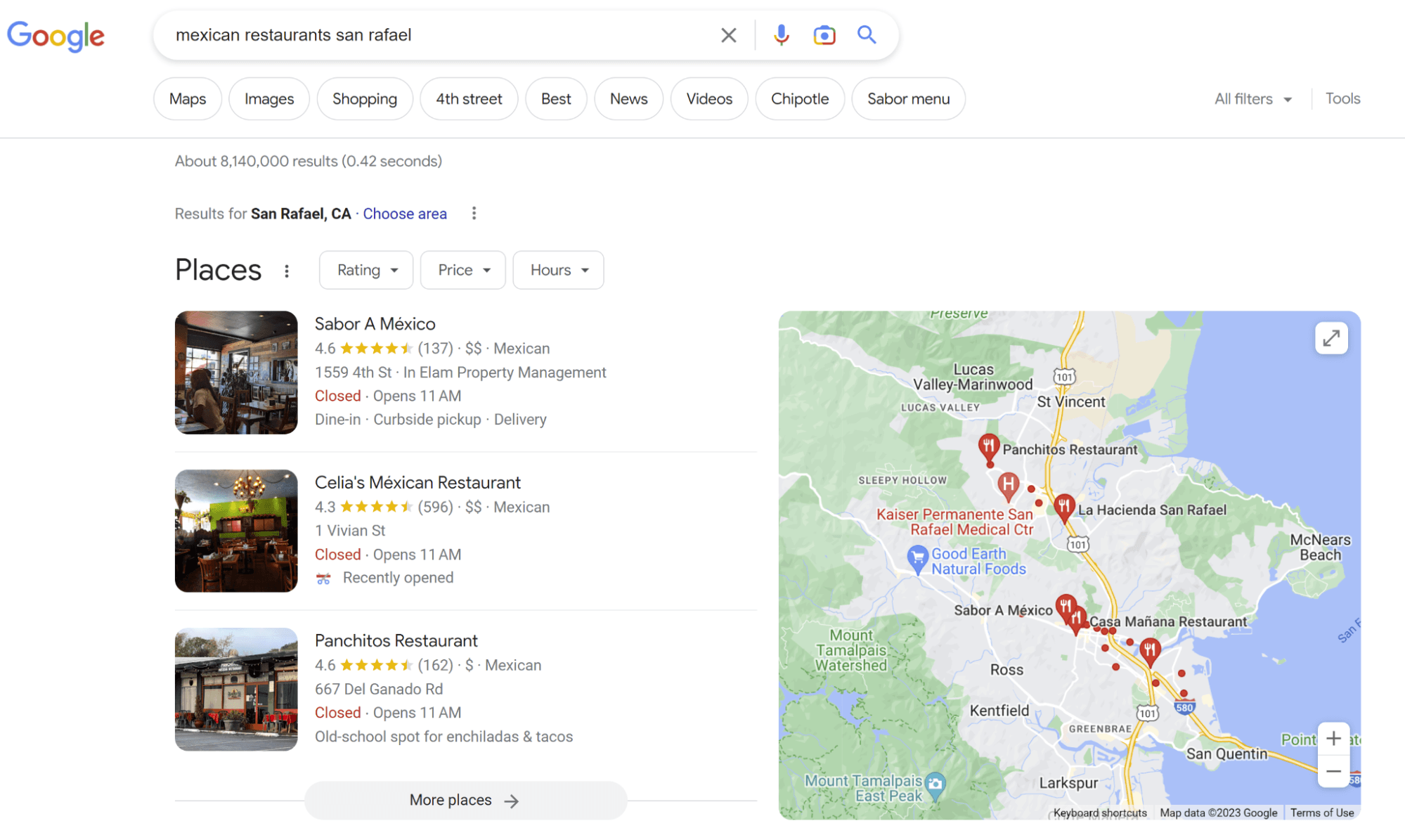A detailed caption for the image could be:

"A color image depicting a Google homepage, showing the search results for 'Mexican restaurants San Rafael.' The Google logo is prominently displayed with its characteristic multi-colored letters in blue, red, yellow, followed by repeating blue, red, and yellow. In the center of the page is the search bar, containing the query 'Mexican restaurants San Rafael.' The search yielded several results in 42 seconds, the first being Sabre a Mexico, rated 4.6 stars. However, it is currently closed and will reopen at 11 am, offering dine-in, curbside pickup, and delivery options. The second listing is for Cecil's Mexican Restaurant, which has a 4.3-star rating. This establishment is also closed, set to open at 11 am, and is a new business in the area. The third result is Pancherito's Restaurant, also rated 4.6 stars and known for its enchiladas and tacos, which will reopen at 11 am. To the right of the listings, a map of San Rafael, California, displays the locations of these three restaurants."